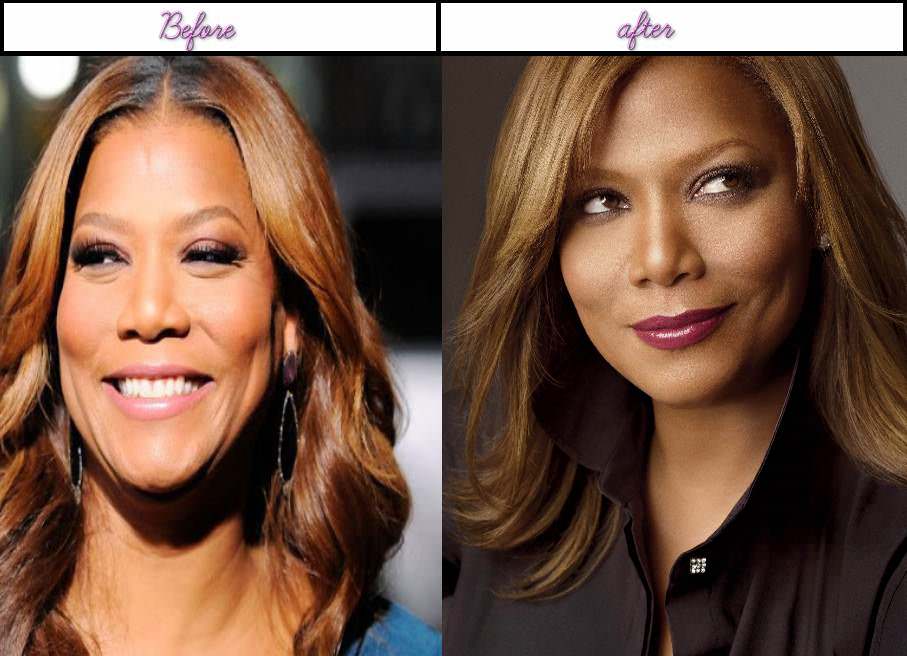The image is a vertically split before-and-after photo of the same woman, featuring two well-spaced side-by-side pictures against a slightly blurred background. The left photo, labeled "before" in purple letters at the top, shows the woman looking slightly to the left. She has long brown hair cascading down both sides of her face, a warm smile, and round earrings. She’s dressed in a blue outfit, visible from the neck up with a glimpse of her shoulder. On the right side, labeled "after," the woman looks slightly to the right. Her brown hair, less curly and cut to shoulder-length, complements her black top with a zipper and a noticeable black collar featuring a small white insignia. She's also smiling, but this time with a closed mouth, and appears to have applied more makeup compared to the "before" image. The overall setting suggests a professional and polished look, indicative of a celebrity before-and-after transformation. The entire image is framed with a thin white border.